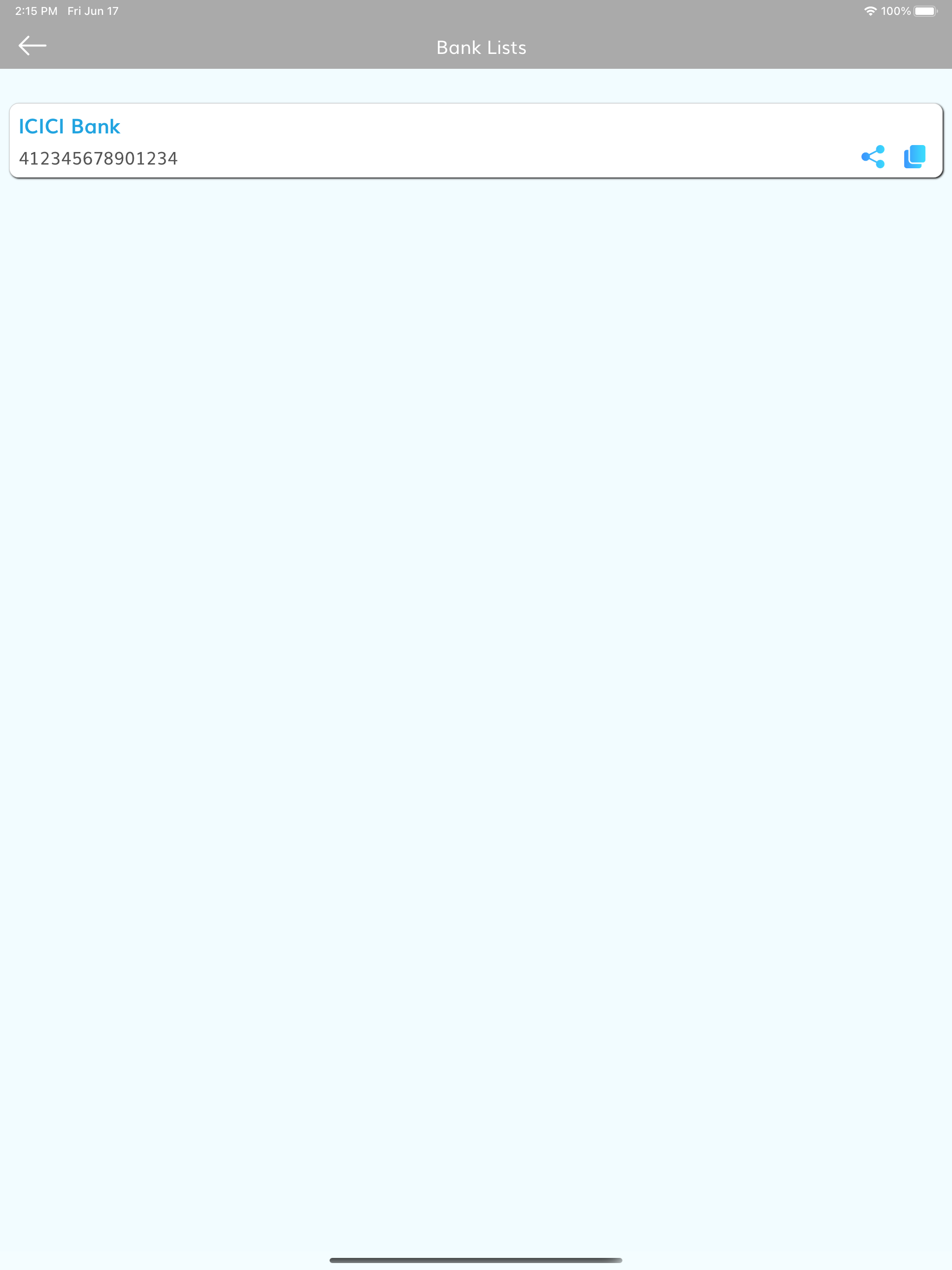A minimalistic screenshot from a mobile banking app is displayed. The app is titled "Bank Lists" at the top, with a clean and uncluttered interface. The primary portion of the screen shows a single entry that reads "I see, I see, I bank," followed by a long numeric sequence, presumably an account number. Below this, there are two interactive buttons labeled "Share" and "Copy," allowing users to share or copy the information. The background features a light, baby blue color, giving the app a soothing visual appeal, while the topmost bar is gray. This top bar contains device indicators such as the notification area, showing a fully charged battery, full Wi-Fi signal, and a timestamp of 2:15 p.m. on Friday, June 17th. Additionally, a back button is visible, suggesting navigational options. The screen is predominantly filled with empty space, emphasizing its sparse and streamlined design, typical of a banking application focused on simplicity and ease of use.